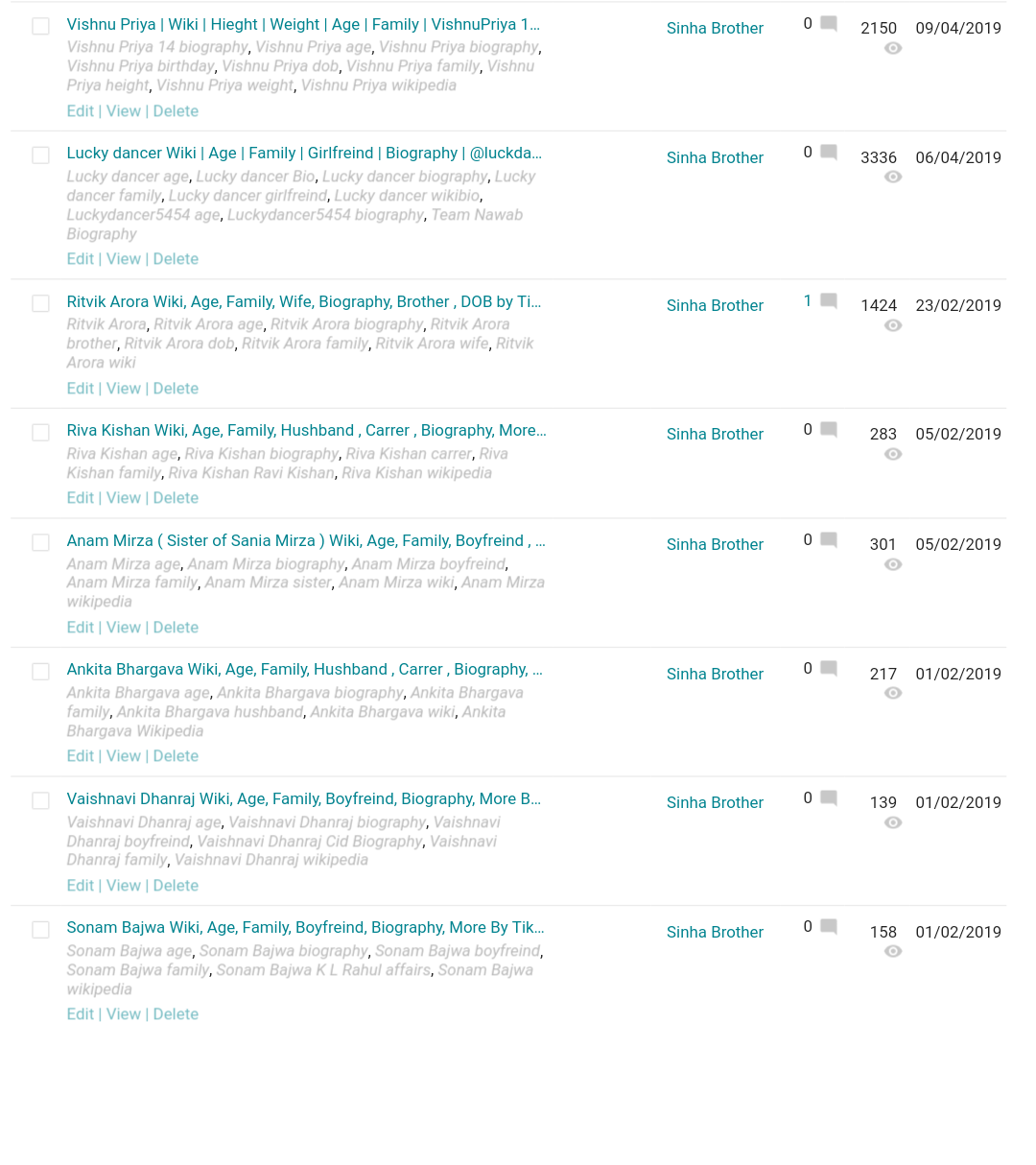The image depicted in the screenshot features a white background with multiple rows reminiscent of notebook paper. Each row is separated by lines and contains various elements in a structured format. To the left of each row is a tickable, transparent checkbox, followed by a light blue text entry.

Each row includes the following:

1. A name, such as "Vishnu Priya," written in blue text.
2. Subsequent entries labeled as "Wiki," "height," "weight," "age," "family," and again, the name "Vishnu Priya" without a space.
3. A repeating phrase "SINHA BROTHER" in blue text.
4. A message icon indicating zero messages for the top entry.
5. A view counter, showing 2,150 views.
6. A date, formatted as "09/04/2019."

This pattern is repeated across several rows, each featuring similar details for different entries.